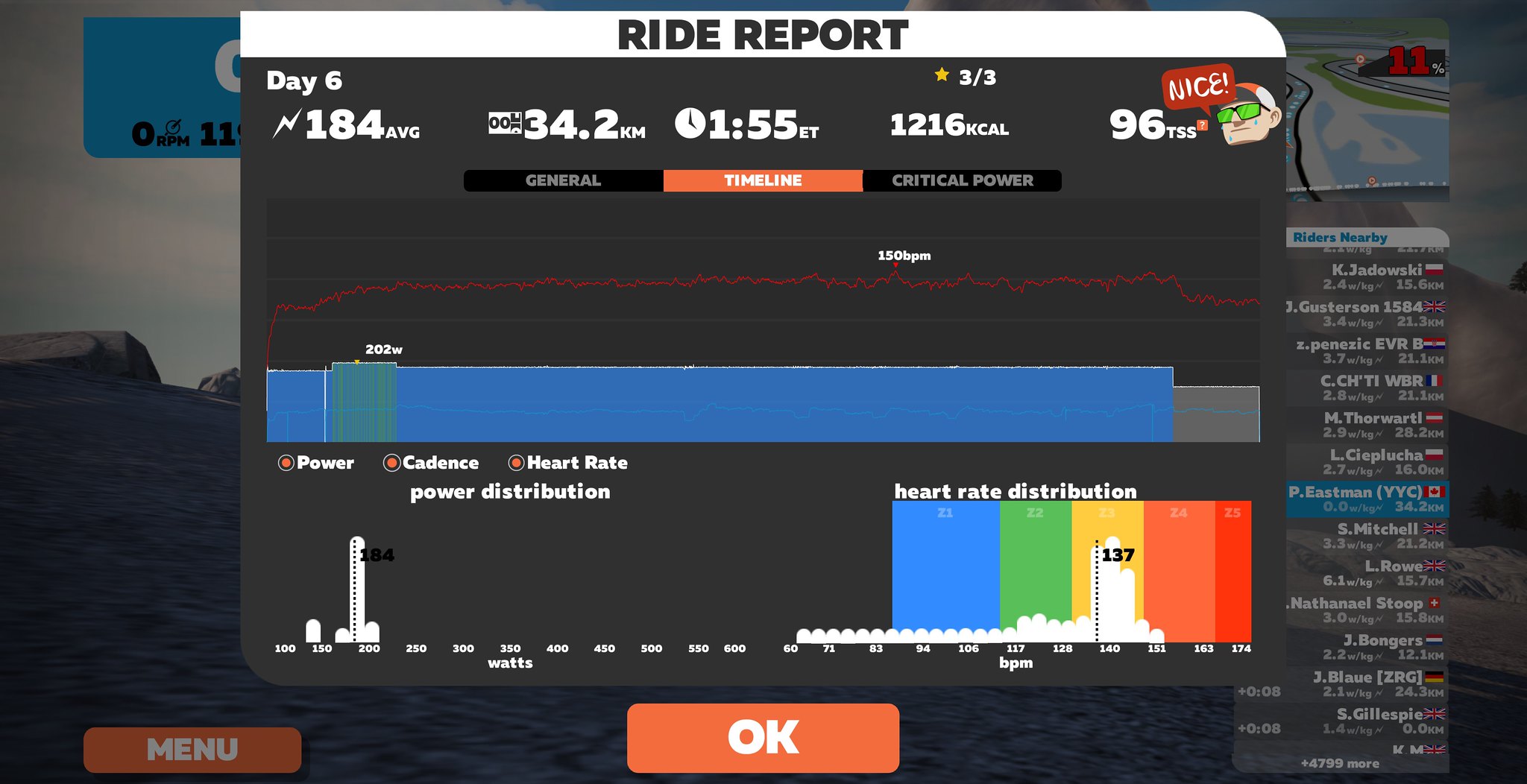The image is a detailed screenshot of an exercise software or video game, focusing on a comprehensive Ride Report. Dominating the center is a large, dark gray rectangle with various data points. At the top, a white, curved rectangle displays the title "Ride Report" in dark gray font. Below, bright white text lists key metrics: "Day 6", "184 average", "34.2 kilometers", "155 ET", "1216 Kcal", and "96 TSS". Further down, three sections labeled "General", "Timeline" (highlighted in orange), and "Critical Power" are separated by a dividing blue bar. A jagged red line graph, presumably showing heart rate data, spans underneath these sections.

The bottom middle of the screen features an orange button with the word "OK" in white text. Towards the bottom left, "Menu" is noted, while the bottom right reveals a multi-colored bar indicating heart rate distribution in a rainbow spectrum. The background includes a secondary image of a water body and other contextual elements such as a "riders nearby" list on the right side and a small map in the top right corner. The overall color scheme is black with accents of white, orange, and blue, providing a structured, analytical view typical of exercise performance summaries.